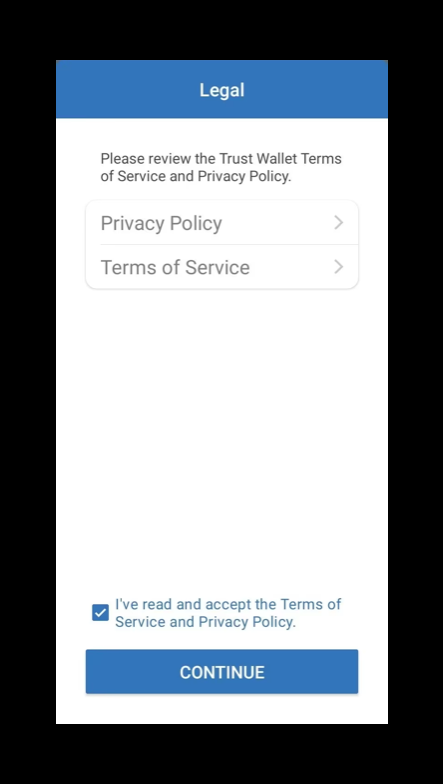A vertical image with a thick, flat, one-dimensional black border encompasses the inner contents. At the top-center of the image, a blue rectangular box displays the word "Legal" in white text. Below this, a white box contains light black text stating, "Please review the Trust Wallet Terms of Service and Privacy Policy." 

Beneath this statement, two grey-bordered rectangular boxes are aligned vertically: the first labeled "Privacy Policy" and the second labeled "Terms of Service," each accompanied by a clickable arrow icon. Toward the bottom of the image, a blue square with a white check mark is present, adjacent to the text, "I've read and accept the Terms of Service and Privacy Policy." At the very bottom, a long blue rectangular button with uppercase white letters reads "CONTINUE."